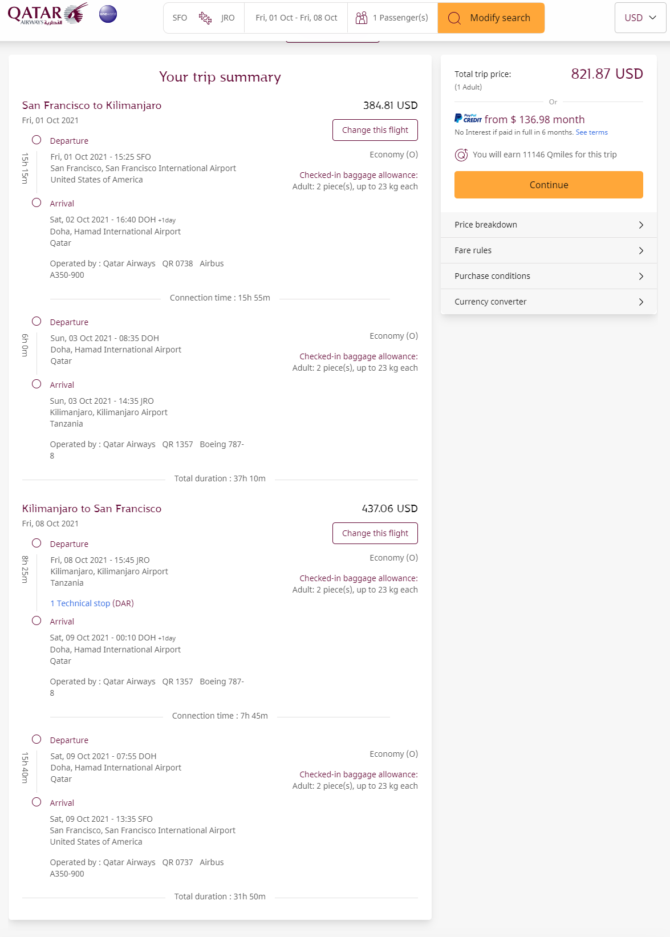**Caption:**

The image showcases a webpage predominantly featuring a booking summary with a white background and burgundy text. At the top, the word "QATAR" is displayed in uppercase letters next to a gray graphic resembling an antelope. Below this, a blue circle with a near-transparent white stripe in the center is visible.

The webpage is divided into various blocks. The first block displays “SFOJRO.” The following block outlines the travel dates: "Fri, 01 Oct - Fri, 08 Oct." The third block specifies "one passenger" with an option to "modify search" highlighted in a yellow-orange color, which is followed by a U.S. state dropdown menu.

Further down, there is a gray-outlined section labeled “Your Trip Summary” in burgundy text:
- Originating flight from San Francisco to Kilimanjaro on Friday, 01 Oct, 2021, costing $384.81 USD.
- Details include departure time, an option to change the flight, checked baggage allowance for adults (two pieces up to 23 kg each), and arrival time.
- Information about connection times and total duration is also provided.

The return flight details from Kilimanjaro to San Francisco are as follows:
- Costing $437.06 USD.
- Includes departure and arrival times, an option to change the flight, and the checked baggage allowance for adults (two pieces up to 23 kg each).